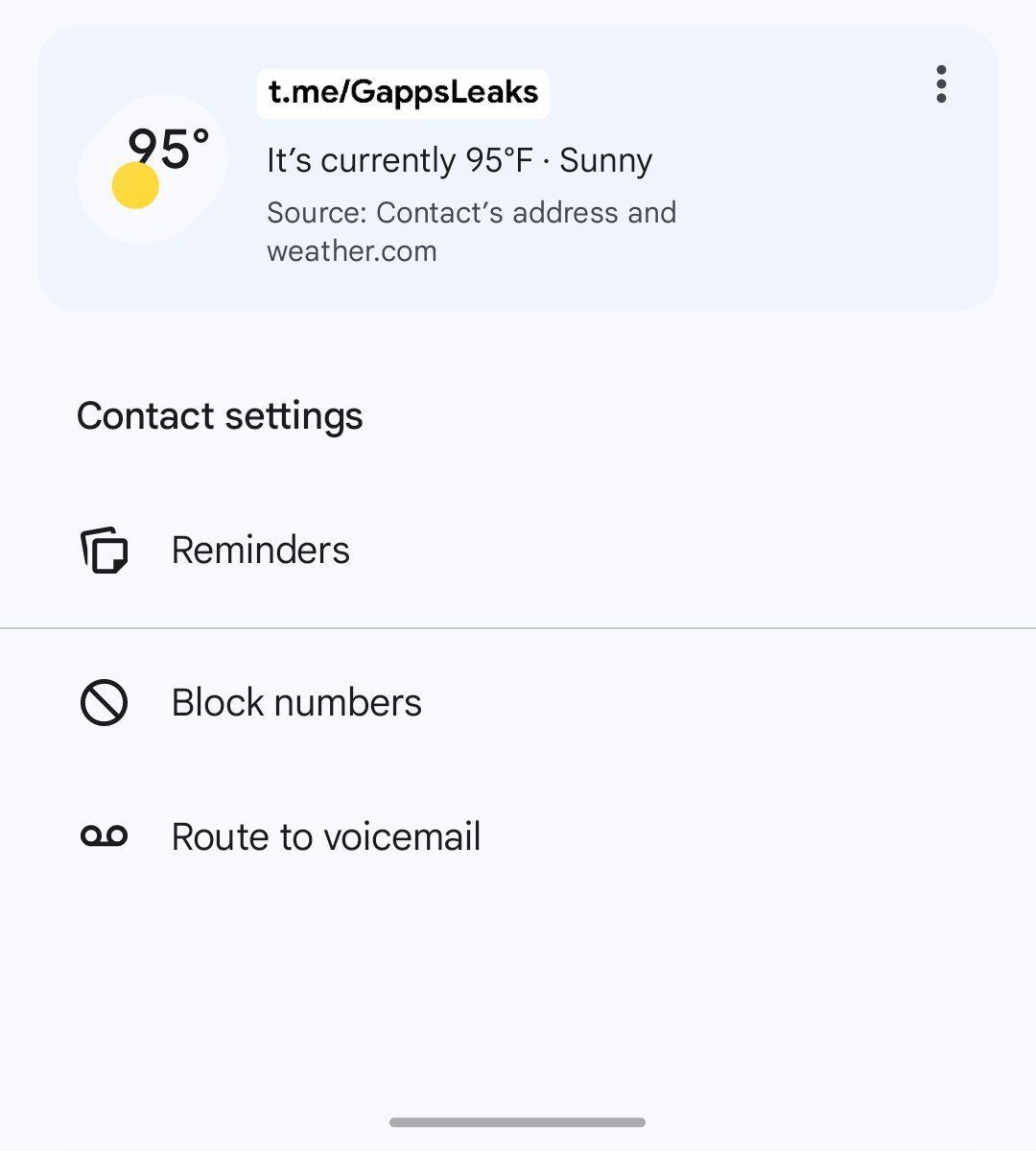This screenshot appears to be taken from a web page or a mobile app interface, showcasing a settings screen with a simplistic and unfinished design. The background is a very pale grey, almost white, setting a neutral tone for the interface.

At the top of the screen, there is a rounded rectangle with a slightly darker grey background that has a subtle bluish hue. Within this rectangle, on the left side, there is a prominent circular icon featuring a yellow inner circle. The text "95 degrees" is displayed next to this icon, along with the link "t.me/gaps_leaks" and three trailing dots on the right side of the rectangle. Below this, the current temperature, "95 degrees" with a "Sunny" status is indicated, along with the source attribution to "contacts address and weather.com."

The main section of the screen lists several options, starting with "Contact Settings" at the top. Each of these options contains an accompanying icon on the left. The "Reminders" option features an icon of two pieces of paper in black and white, followed by "Block Numbers" which has a circle with a line through it, indicating blocking functionality. The last option, "Route to Voicemail," is represented by a tape icon.

There is a thin grey line separating each option, providing subtle delineation between them, although it is particularly noticeable between "Reminders" and "Block Numbers."

At the bottom of the screen, there is a small, greyish horizontal band that spans about a quarter of the way across the width of the screen, positioned in the center. 

Overall, the interface gives the impression of being a template or a work-in-progress, possibly a prototype for a mobile settings screen or a web interface, rather than a finished, polished product.